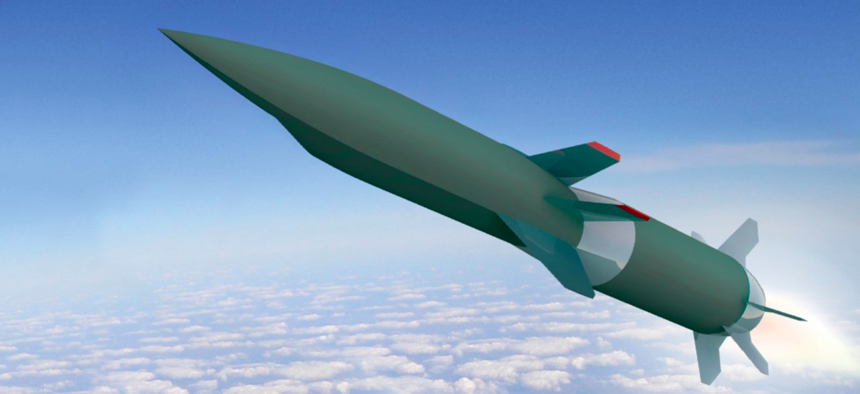This is a detailed image of a cartoonish, three-dimensional rocket soaring high above a scattered, cloudy sky. The sky features a gradation from pale blue at the bottom third, transitions through a strip of hazy white clouds in the middle, and becomes bright blue at the top. The rocket, appearing in pale olive green, has a sharp needle-like tip positioned near the top left of the frame. This tip curves back towards a teal blue fin adorned with a red stripe at its tip, which meets a silver cone section. The rocket body includes another segment of olive green cylinder, and the darker green bottom part is separated from the olive green section by a straight line. At the rear end, five silver, reflective fins are visible. A white teardrop-shaped flame, tinged subtly with orange at its core, emanates from the rocket's base in the bottom right corner of the frame. The sky background, with its scattered clouds below and ethereal wisps, highlights the animated nature of the rocket.